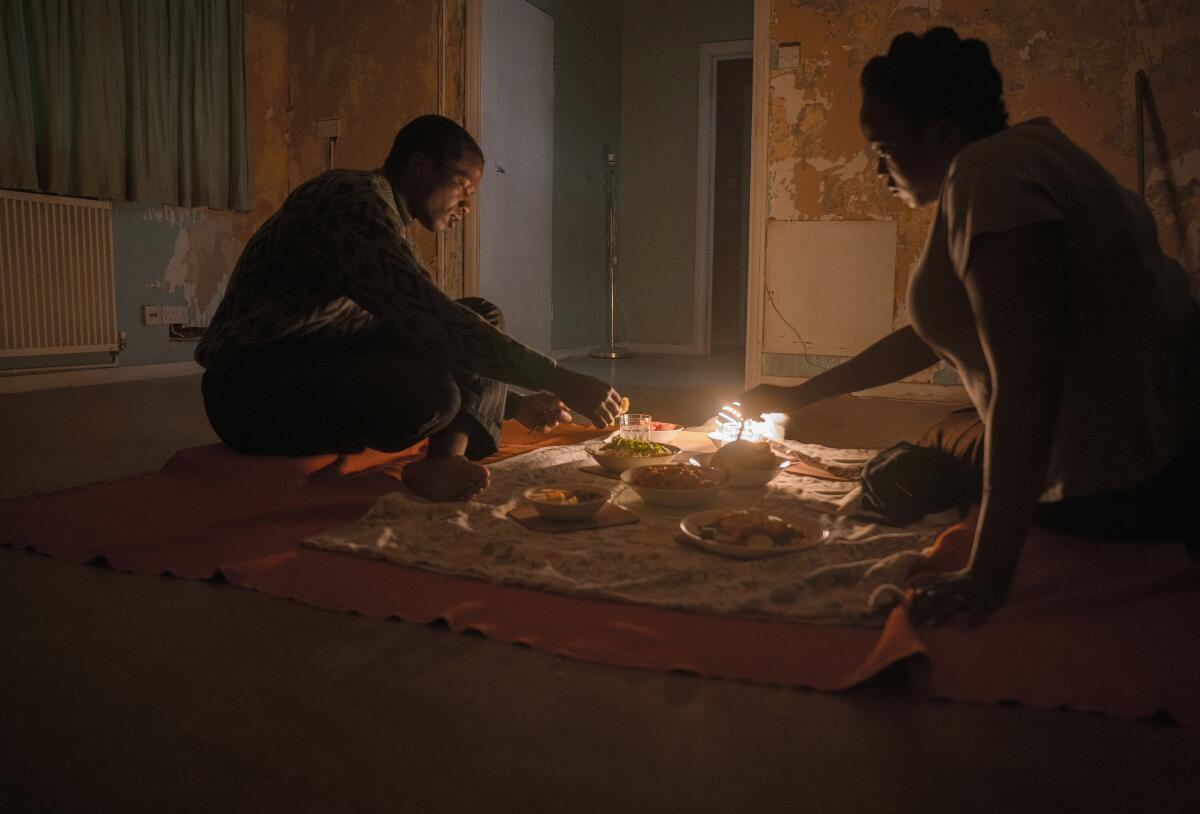In a scene from the movie "His House," a black couple is depicted sitting cross-legged on a worn blanket inside a sparsely furnished room, sharing a meal placed on a mat and napkin on the floor. The man on the left is dressed in a tan and brown sweater with black and white pinstriped trousers, while the woman on the right, partially obscured by shadows, is wearing a tan shirt and brown pants. The room around them is dilapidated, with yellow walls marred by peeling paint revealing white patches, hinting at the building's age and neglect. A white socket and a white vent, likely an air conditioner, are visible on the left side, beneath green curtains. Two white door frames stand in the background, with one door slightly ajar. The scene is lit by a floor lamp, casting a stark light that heightens the ominous atmosphere. The wooden floor, covered in places by the blanket, adds to the room's rundown appearance, and various plates and bowls filled with food such as green, yellow, and brown dishes, and cucumbers are arranged around the couple, along with clear glasses. A silver post with a white light bulb stands in the left corner, contributing to the eerie vibe of this poignant moment from the film.